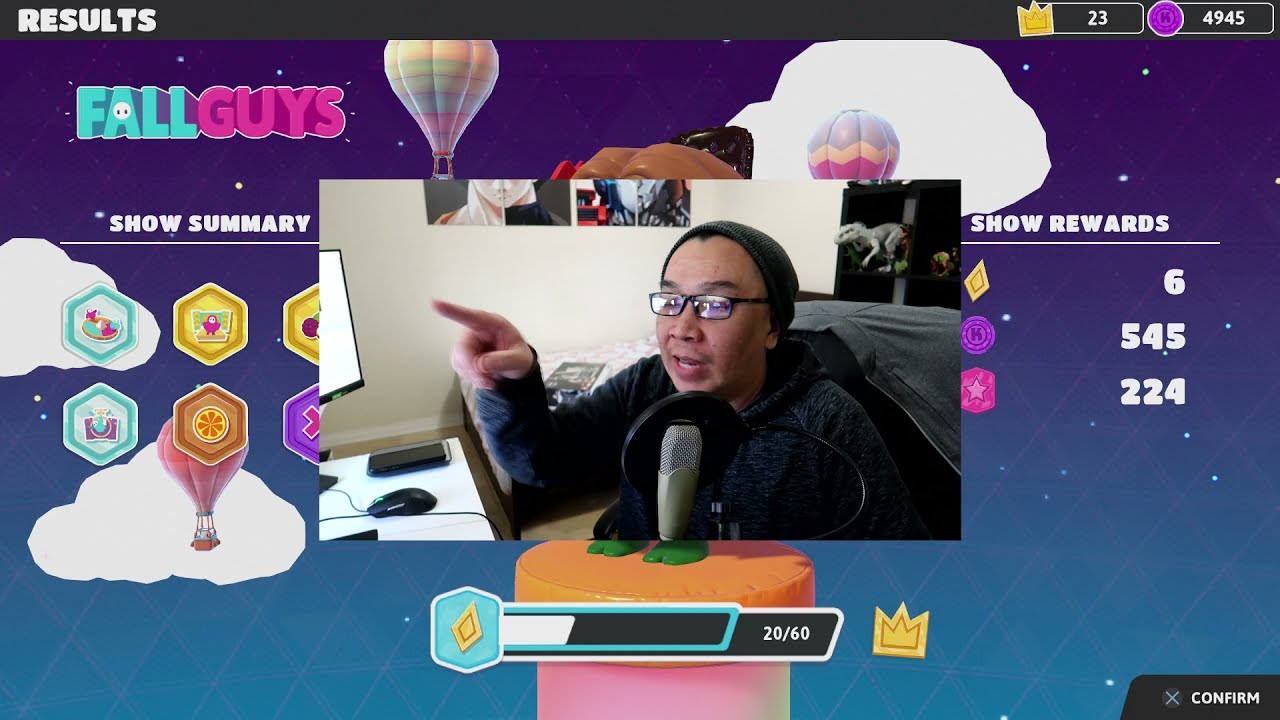The image features an inset photo of an Asian man live streaming from his bedroom, superimposed on a "Fall Guys" video game menu screen. The man is seated at a desk, pointing towards his computer monitor with his right hand while speaking into a gray metal microphone topped with a black windscreen. He has black-framed glasses, a black beanie, and is wearing a black sweatshirt. Behind him, you can see a chair with a jacket draped over it and a few pictures on the wall. The desk holds a computer screen, a mouse, and a cell phone. The "Fall Guys" interface shows a blue to purple gradient background, with text in the upper left corner reading "Fall Guys." Below that, "Show Summary" is visible, and to the lower right, it says "Confirm" with an X. Additional elements include a hot air balloon icon, a results bar reading "20 out of 60," and an achievement bar at the bottom.